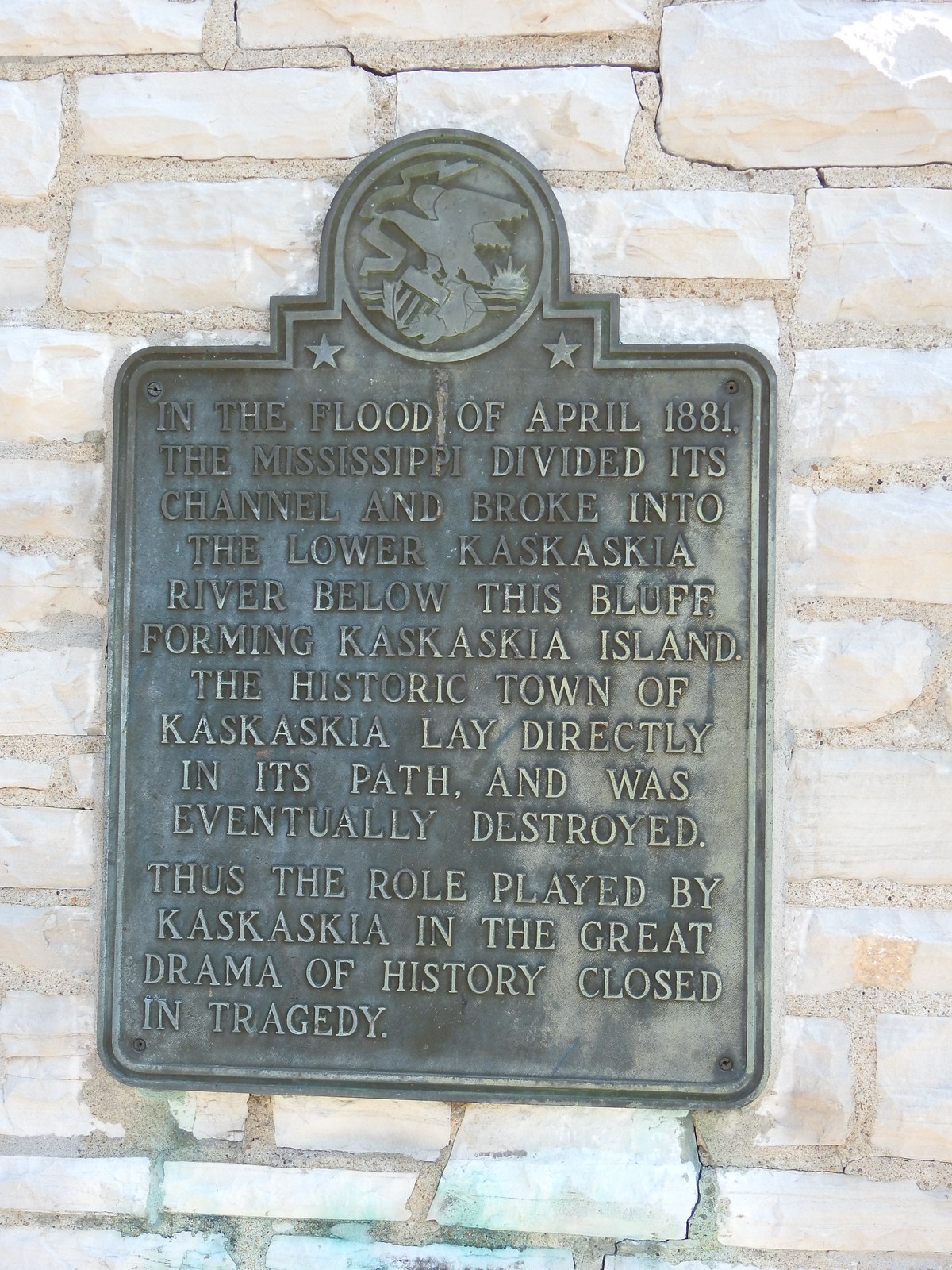The image depicts a historical plaque mounted on a white and light brown uneven brick wall. The plaque, appearing to be made of a dark greenish metal, bears a detailed insignia at the top. This insignia features a bird, presumably an eagle, holding a white ribbon in its mouth with a setting sun in the background and a shovel-like object in front of it. The plaque is adorned with a star in each corner of the circle housing the bird. 

The inscribed text reads: "In the flood of April 1881, the Mississippi divided its channel and broke into the lower Kaskaskia River below this bluff, forming Kaskaskia Island. The historic town of Kaskaskia lay directly in its path and was eventually destroyed. Thus, the role played by Kaskaskia in the great drama of history closed in tragedy."

Overall, the plaque serves as a solemn reminder of the historical events that led to the destruction of Kaskaskia, marked by the symbolic imagery and detailed account of the fateful flood.